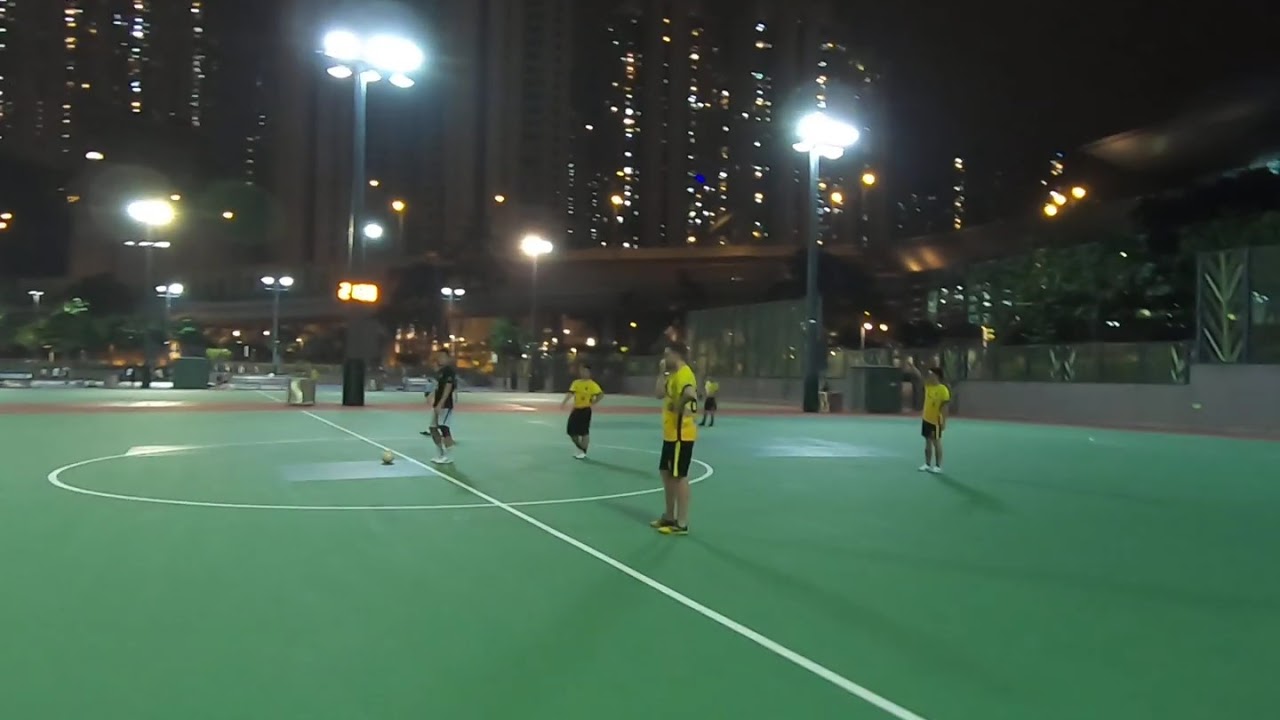The image is a vivid nighttime photograph of an urban soccer field with a landscape orientation. The soccer field, which is covered in bright artificial green turf and marked with solid white lines, features a central circle dissected by a line extending towards the horizon. The scene is illuminated by multiple floodlights positioned along the edges of the field, casting a stark light on the players and the vibrant green turf.

Visible in the foreground are several soccer players, predominantly gathered to the right side of the central line. The players are distinguishable by their matching yellow jerseys paired with black shorts and either yellow or black sneakers. Some sources suggest there might be about a dozen players in total while others specify five or six are distinctly visible.

Surrounding the field is a divider wall with a solid cement or stone base topped with glass, ensuring a clear view into the playing area. In the background, the expansive city skyline is illuminated by numerous towering apartment buildings, suggesting the urban environment in which this field is situated. Despite the apparent isolation of the scene, the background highlights the bustling, lively city at night with its multitude of lit windows.

The image appears to be captured from a viewpoint akin to a stadium seat height, possibly through a drone, providing a comprehensive view of both the field and the surrounding urban landscape. The detailed composition and photographic realism emphasize the contrast between the illuminated field and the darker cityscape beyond.